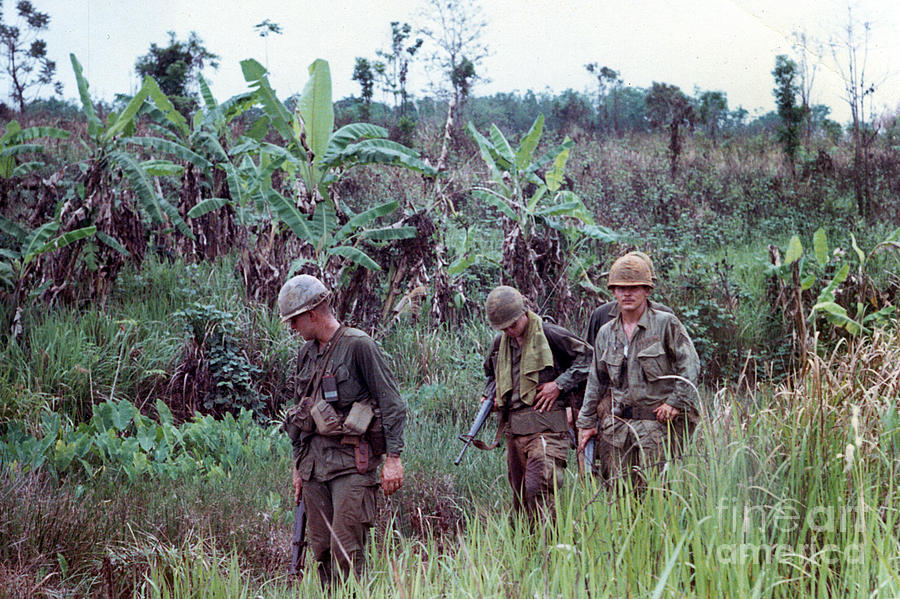In this photograph, four American soldiers, appearing to be in their early 20s, traverse a high brush plateau with a tropical, Southeast Asian feel, likely Vietnam. Dressed in dark green combat fatigues and standard helmets, the soldiers carry rifles and belts equipped with canteens. They walk in a line, with one soldier slightly behind the others, their expressions relaxed and focused downward, as if scanning the terrain. Among them, the second soldier is distinctive, with a lighter green towel draped over his neck. The backdrop features spaced-out tall trees, shorter palm or banana-like trees, and tall grass, all under a gray, hazy sky. The text "Fine Art America" is subtly visible in the bottom right corner, adding an artistic touch to the historic scene.